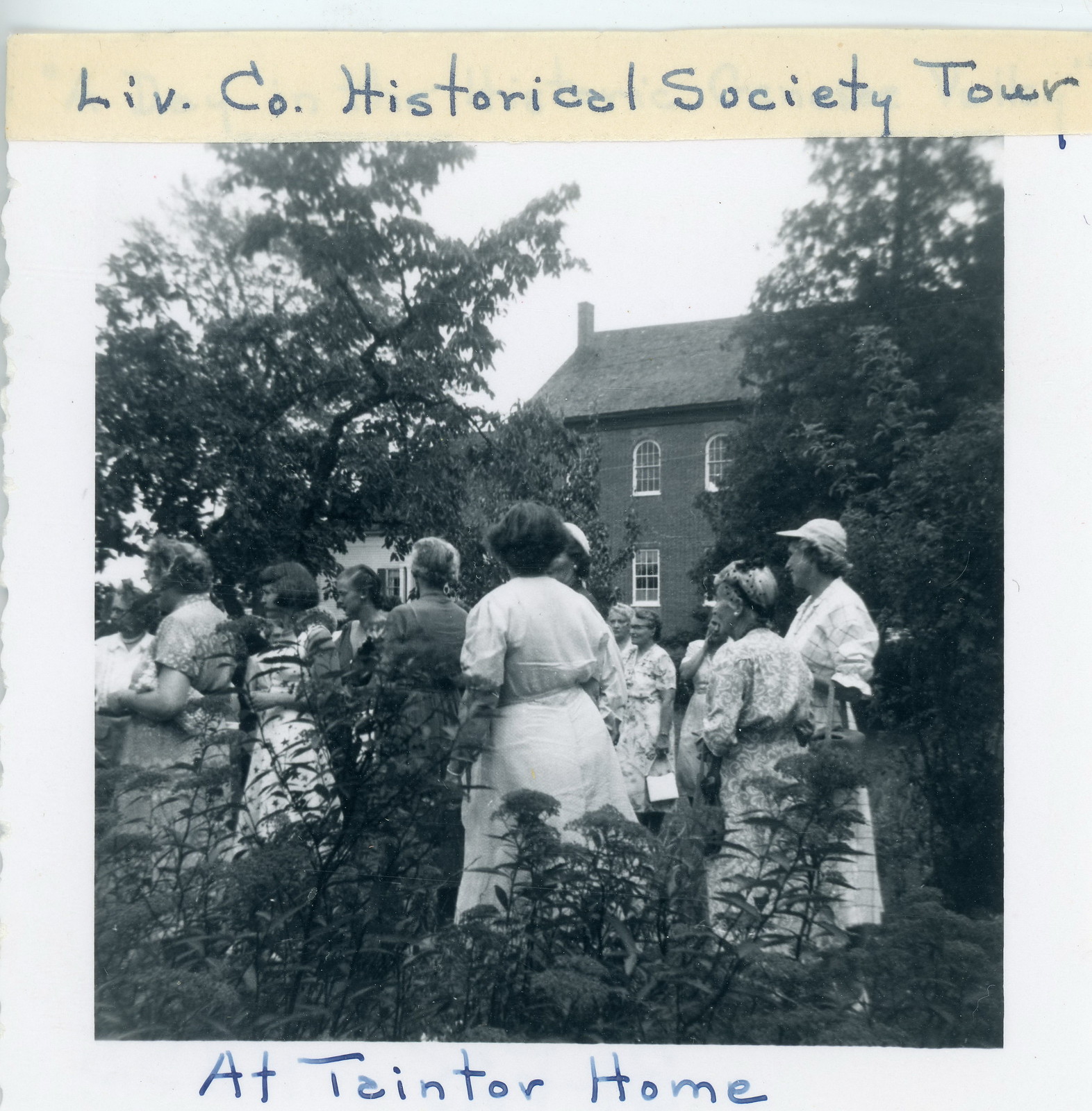This black and white historical photo is bordered by a white frame, with a piece of masking tape at the top inscribed in blue ink with "LIV. co. historical society tour." The caption "At Tainter Home" is similarly written on the bottom white border. The image, possibly dating from the late 1940s or early 1950s, features a group of women dressed in an array of dresses, some wearing hats and holding purses. These women are gathered in front of a large, multi-story brick building that is partially obscured by trees and has a prominent roof. In the foreground, overgrown weeds or flowers slightly obscure their lower bodies, adding an element of depth. The photo captures a moment from a historical society tour, with the women appearing to engage in conversation or await the next part of the event.